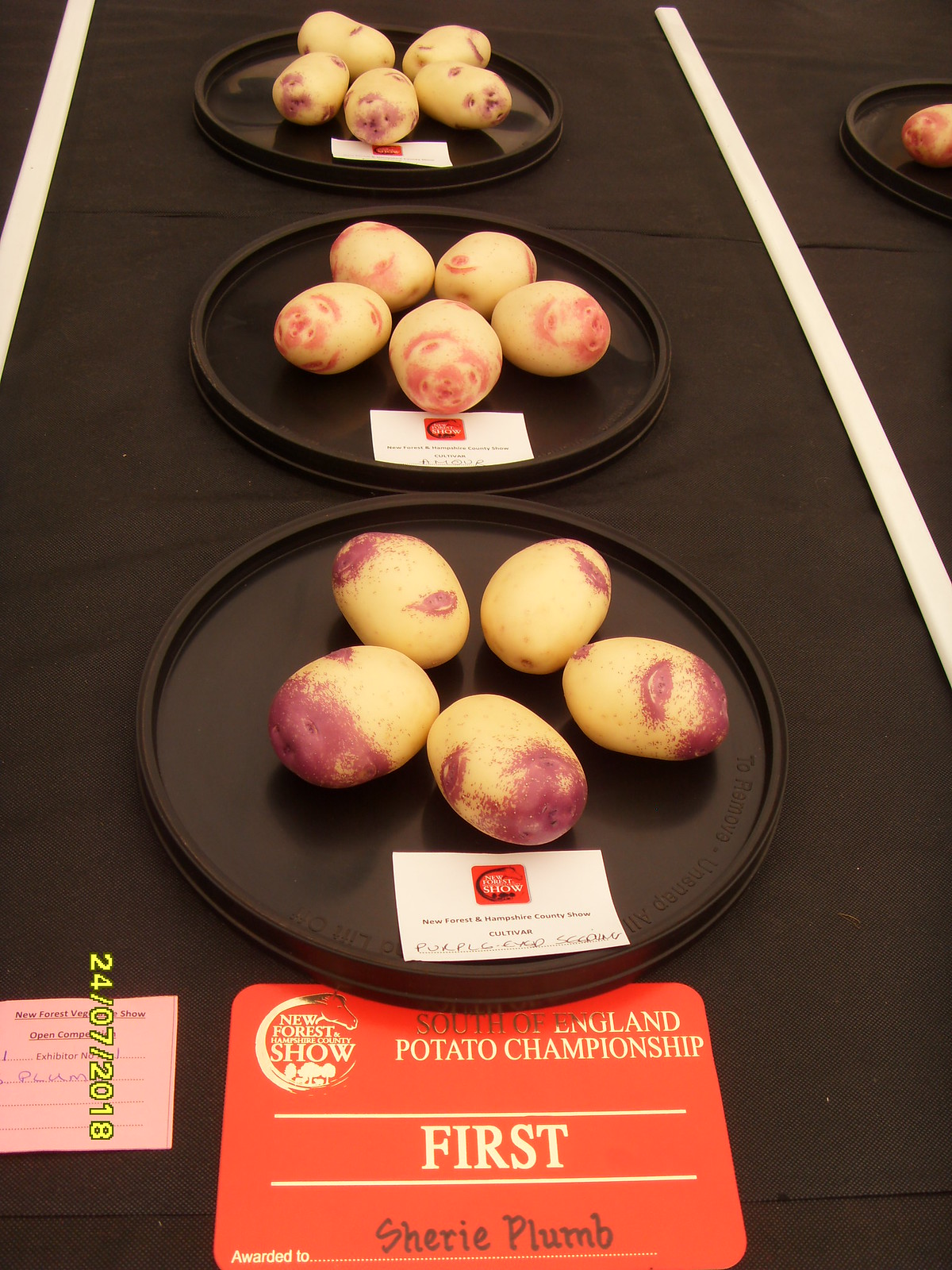The image depicts a cooking competition, specifically the South of England Potato Championship at the New Forest Show. At the forefront is a large table adorned with a black tablecloth featuring white borders. Arranged on this table are multiple black, circular plates, with the primary focus on three centered plates, each holding five potatoes. 

The potatoes vary in color, including purple and yellow varieties. The middle plate prominently features a certificate that reads "South of England Potato Championship," awarded to Sherry Plum for first place. The certificate features the New Forest in Hampshire County Show logo, which includes a circular emblem with a horse and trees.

Beside these plates, there is also a pink form and a partially visible yellow date stamp "24-07-2018." In addition, the upper corners of the image show other participants' entries bordered by white vertical stripes. The overall scene showcases the competitive arrangement and proud display of Sherry Plum's award-winning potatoes.